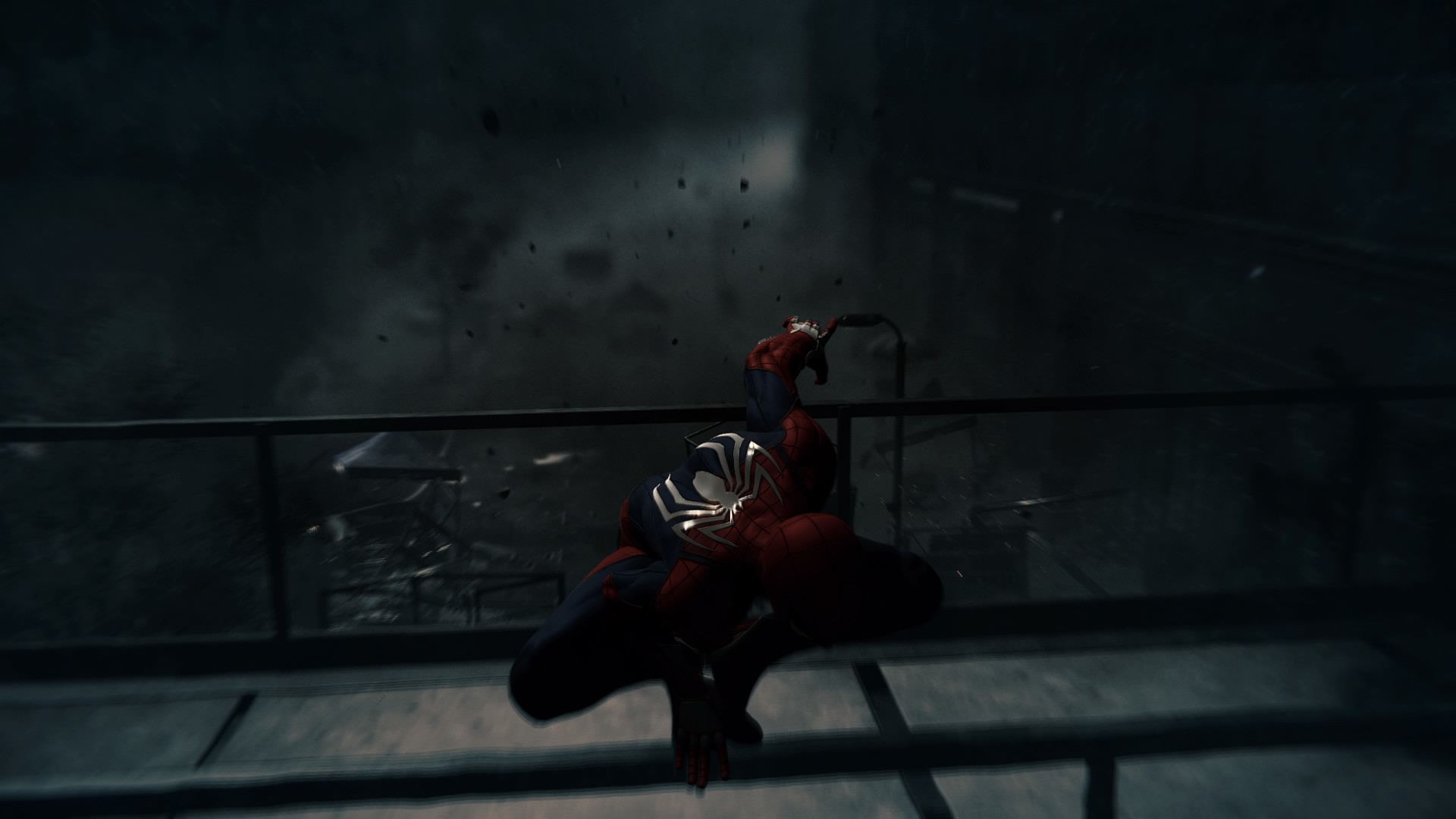In this screenshot from a Spider-Man video game, Spider-Man, clad in his iconic red and blue suit with a silver spider emblem on his back, is striking a dynamic pose on a steel platform or railing in what appears to be a warehouse. He is crouched low with both feet together, knees bent deeply, and his back contorted in a dramatic fashion. One hand touches the floor near his feet while the other is stretched out behind him. The environment around him is chaotic, with debris and smoke in the air, suggesting a recent explosion or intense conflict. The setting includes gray walls and exposed rafters near the ceiling, adding to the industrial atmosphere of the scene.